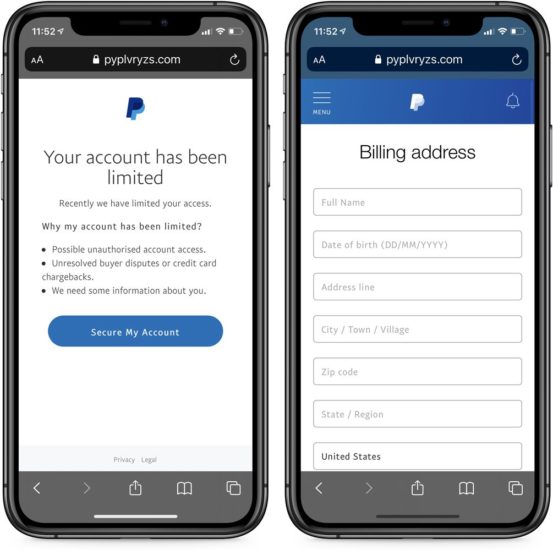In the image, there are two smartphones displayed side-by-side. The phone on the left shows a warning message indicating that the user's account has been limited, highlighting potential reasons such as unauthorized access, unresolved buyer disputes, or credit card chargebacks. The interface prompts the user to provide information to secure their account, featuring navigational elements like a back arrow, forward arrow, upload button, bookmark, copy icon, privacy policy link, and a legal notice, all encompassed by a distinct white line.

On the right, the other phone screen prompts the user to enter their billing address details, including full name, date of birth in the DDMMYYYY format, address line, city/town/village, zip code, state/region, and country (United States). Similar to the left phone, this screen also includes a back arrow, forward arrow, upload button, bookmark, copy icon, and a black line, emphasizing the importance of inputting personal information to secure the account. The UI elements are consistent, mirroring those on the left phone screen, ensuring a seamless user experience.